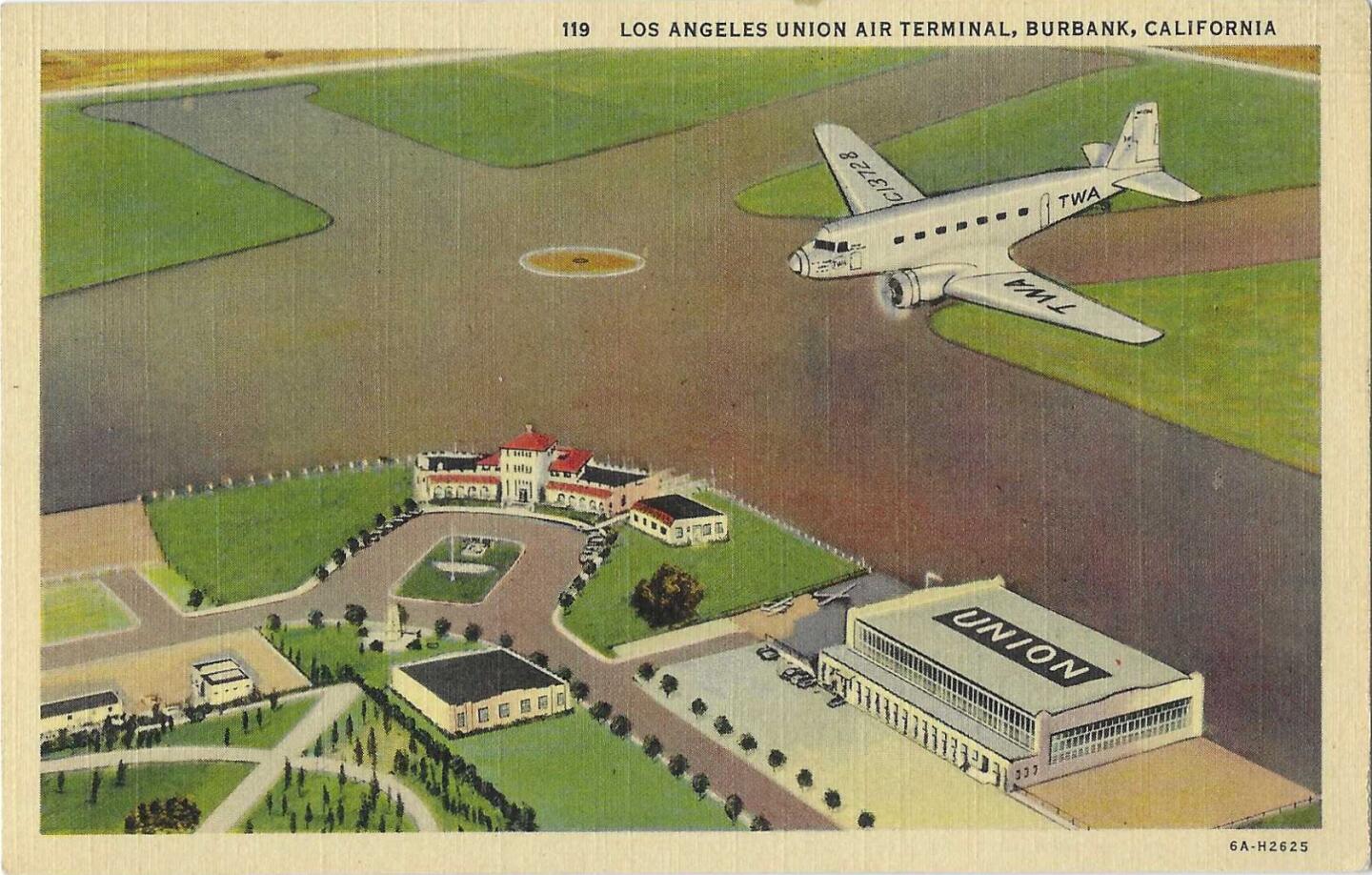The image is a vintage colorized illustration, resembling a postcard from the 1950s or 1960s, depicting a small propeller plane with "TWA" (Trans World Airlines) stenciled on its wing and tail, approaching the Los Angeles Union Air Terminal in Burbank, California. The plane, positioned in the top right corner, is descending towards an intersection runway that extends in an ellipse from the top left to the bottom right of the image. The vibrant illustration utilizes a palette of green, lime green, white, black, red, orange, brownish-greenish, and purplish-reddish hues. Below the plane in the detailed landscape, various airport buildings are visible. Centrally, there is a long, two-story white terminal with a red roof. To its right stands a more modern hangar facility with a flat roof, labeled "Union" in bold white text on a black background. The top right corner of the illustration is bordered by the text "Los Angeles Union Air Terminal, Burbank, California", although some additional text at the bottom right is illegible. The detailed architectural elements and vintage style suggest that this scene is a realistic depiction of the era's bustling air travel hub.